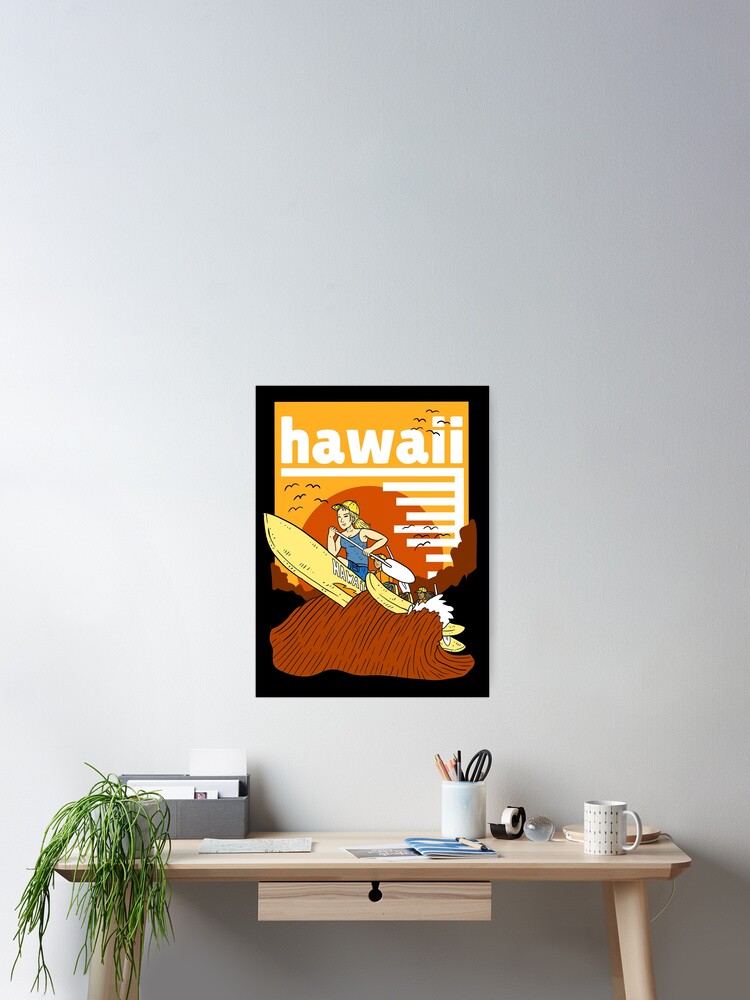This is a vertical rectangular photograph of a small, modern, light beige wooden desk against a mostly bare, gray wall. The desk, which has one central drawer equipped with a black key lock, stands on four slim legs. On the left side of the desk, there is a lush green plant with leaves cascading down, partially obscuring a vertical file holder behind it. The desk is adorned with several items: a white mug filled with pens and scissors, another empty white coffee mug, loose papers, a blue booklet, and a black tape dispenser with clear tape. Positioned on the back-right corner of the desk is a white, flexible desk lamp angled down to illuminate the workspace. Above the desk hangs a framed picture depicting a surfer on a yellow surfboard, riding a red wave against a backdrop of a vivid sunset and yellow sky. The picture, bordered in black, features the word "Hawaii" in lowercase white letters. Notably, the floor and a chair are not visible in the image.